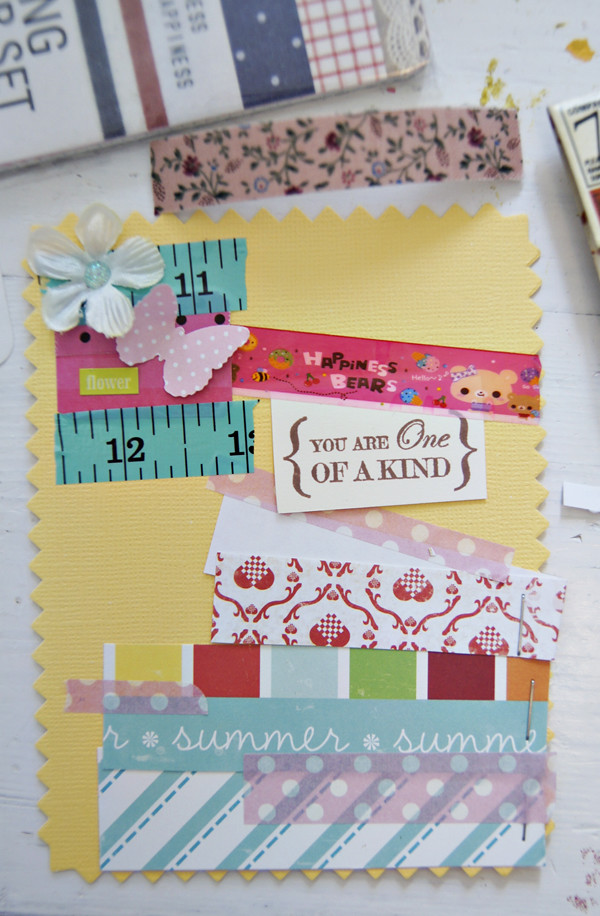The image captures a bright and clear scene of a white-painted wooden table adorned with various arts and crafts supplies. The centerpiece is a yellow card, intricately bordered with a rounded triangular cut-out pattern. This card is decorated with various strips of paper, each showcasing unique designs. One strip features ruler markings, while others boast images including bears labeled "Happiness Bears," and a strip displaying the phrase "summer summer" in white text against a blue backdrop. Above these, a multicolored strip is adorned with a red heart design. On the upper left of the card, there's a white flower with a blue center next to a pink polka-dotted butterfly. The middle right part of the card bears a significant message that reads, "You are one of a kind."

In addition to the central card, the table hosts additional embellishments. There is a pink strip with flower designs, situated above the arts and crafts display, featuring flowers in shades of pink, red, blue, and light blue. A piece of packaging, featuring red and blue stripes with four white dots, is visible on the upper left. The scene is naturally lit, enhancing the vivid colors and details of the crafted elements, creating a cheerful and vibrant atmosphere.